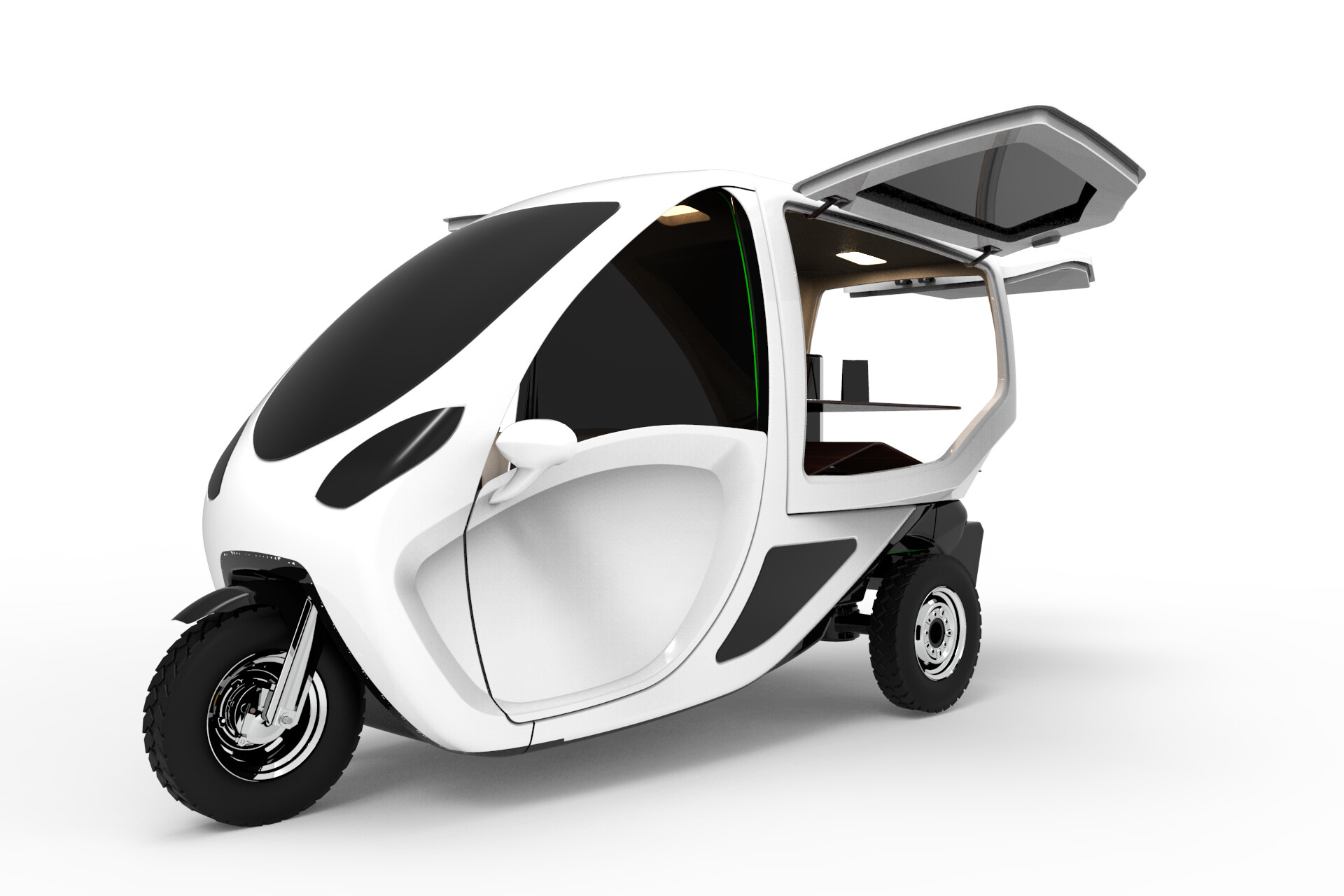This image depicts a futuristic, high-tech, three-wheeled vehicle that is primarily white with black tinted windows. The vehicle has one wheel in the front and two in the back, with silver rims adorning the black wheels. The design features a sleek, curved windshield and a pod-shaped door on the side, which is propped open to reveal the interior. Inside, there is a shelf or table holding a black object and a cup, indicating storage capabilities.

The vehicle's small, bubble-like structure suggests it is designed for a single occupant. It has glossy, dark-tinted windows all around, providing privacy and a modern aesthetic. Both the door and the rear compartment are open, allowing a clear view inside. The front of the vehicle showcases distinctive headlights, giving it an almost "eye-like" appearance, and side mirrors are mounted on the exterior. The front wheel is supported by a chrome assembly, enhancing its futuristic look. The overall impression is of a compact, innovative vehicle, possibly a concept model, blending elements of a scooter, a golf cart, and a small car.